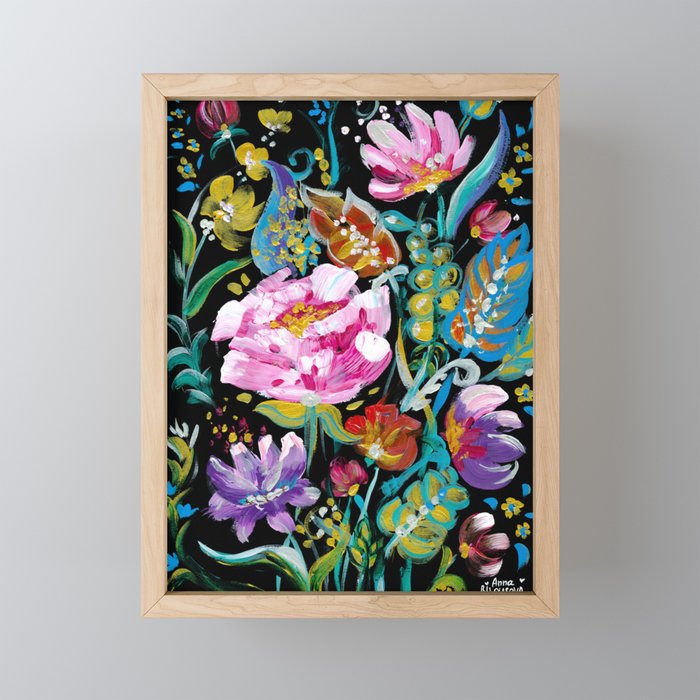This image is a color photograph depicting a framed, vibrant floral painting by an artist named Anna, although the frame cuts off her last name. The frame is made of simple light wood, which contrasts with the piece. The canvas is rectangular and oriented in portrait style against a gray wall. The entire background of the painting is solid black, creating a striking backdrop for the brightly colored flowers. These flowers include purples, various shades of pink, deep blues, sea greens, and turquoise leaves, along with small yellow flowers that have either white or turquoise accents and dark pink dots. The painting exudes texture, potentially due to oil painting techniques, with evident brush marks adding depth. The artist's signature, "Anna," is located at the bottom, accompanied by two hearts.